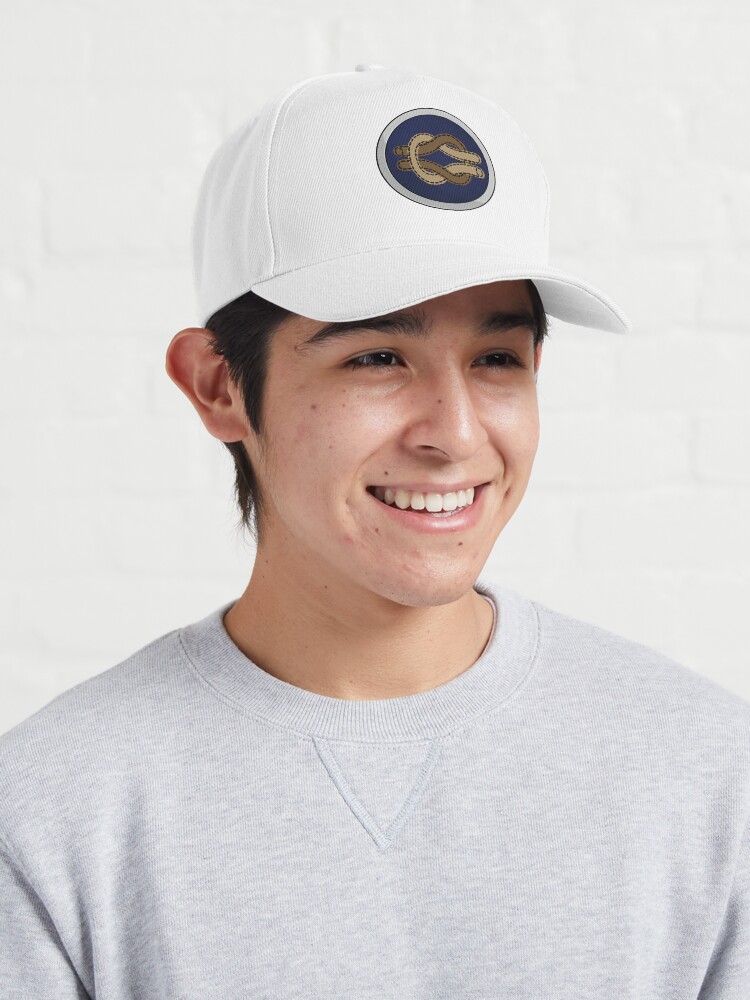The image features a young smiling Asian male, who exudes a warm, albeit slightly posed, expression. He is dressed in a light gray, jersey-knit sweatshirt with a crew neck collar, notable for its V-shaped seam at the center of the collarbone. His short hair is partially visible, with sideburns extending to his ears and some hair trailing down the back of his neck. 

Topping off his look is a solid white baseball cap adorned with a distinctive circular logo. This logo is composed of a silver outer circle and a black background featuring a knot in the center, resembling a square knot with one half in light tan and the other half in a whiter shade. The man's dark eyebrows, light brown skin, and slightly squinting eyes further emphasize his engaging smile.

Against a backdrop of a well-lit white brick wall, the photo is overall bright, filled with natural daylight illuminating his face, enhancing his features, and making the environment feel welcoming.